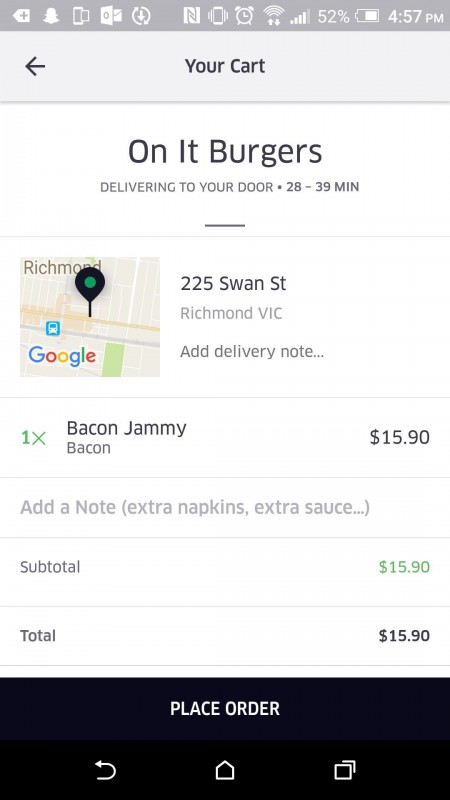This is an image of a smartphone screen displaying a food delivery app. At the very top, on a dark green-brown status bar, various icons are visible: the Snapchat symbol, a phone symbol, fragmented squares, a circle, a large "N" indicating NFC, a vibrating phone icon, a clock icon, a Wi-Fi symbol, signal bars, and a battery icon showing 52% at 4:57 PM.

Below the status bar, a map interface is displayed in shades of green and gray, indicating the user's car position and a left turn. The screen shows an order for burgers with estimated delivery time between 28 to 39 minutes to the address 225 Swan Street, Richmond, VIC. The screen further specifies options to customize the order, including adding "reno" and selecting add-ons such as bacon jammy bacon for $1.1590, alongside fields to add notes for "extra napkins" and "extra sauce." The subtotal and total both amount to $1.1590, with the option to "Place Order" shown below. At the bottom, there are icons resembling a house and squares.